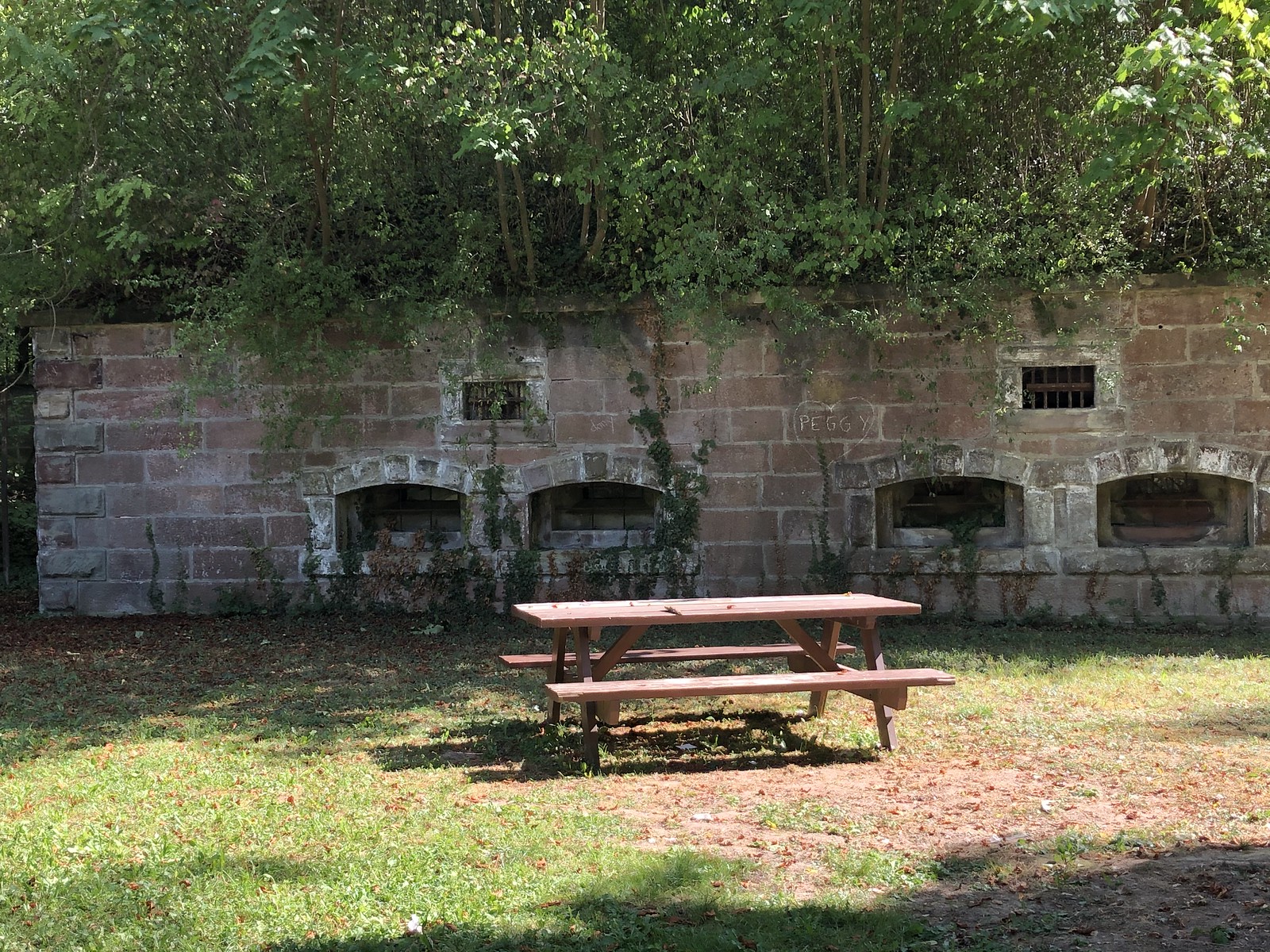A detailed image of an outdoor park features a tan wood picnic table with attached benches situated slightly to the bottom right of the frame. The table rests on a patchy courtyard where the grass is sparse and vividly green on the left but more barren towards the bottom right. Looming in the background is a tall brick and concrete wall, described as a mix of reddish-tan tones with gray and brown bricks that line several architectural features. This wall has multiple rectangular holes—four large arches grouped in pairs at the bottom and a smaller, grate-covered rectangle positioned above them.

Behind and above the wall, the scene transitions into a deeply wooded area filled with lush, thick trees and heavy foliage. Vines and ivy drape over the wall, adding to the sense of overgrowth. The shadows of other unseen trees stretch across the scene, adding contrasting patches of light and shade. The overall setting exudes a sense of rustic tranquility, enhanced by the abundant greenery and the interplay of shadows and sunlight.